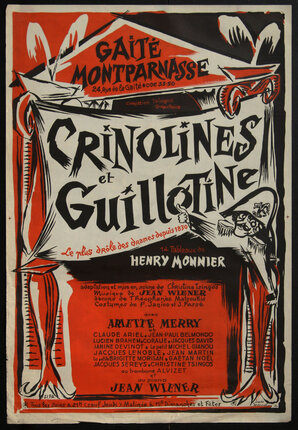The image is of an old theatrical poster framed by a thin black border. It depicts a stage setting with side curtains and a red-tinted tent at the top, reminiscent of a stage or circus tent. At the very top, within the tent, "GAI-TE MONTPARNASSE" is written in bold black letters. Below this, a wide white banner spans the width of the poster, displaying the text "CRINOLINES ET GUILLOTINES" in large black print. There is a small illustration of a French officer to the right, adorned with a traditional uniform that includes shoulder tassels and a Napoleon-style hat. Beneath the banner, against a black background, "Henry Monnier" is prominently displayed in white letters. The bottom section of the poster features a red background with several lines of small black text, which includes names like "Mary" and "Jean Wiener." The entire poster is designed with tones of red, black, and off-white, giving it a vintage appearance.